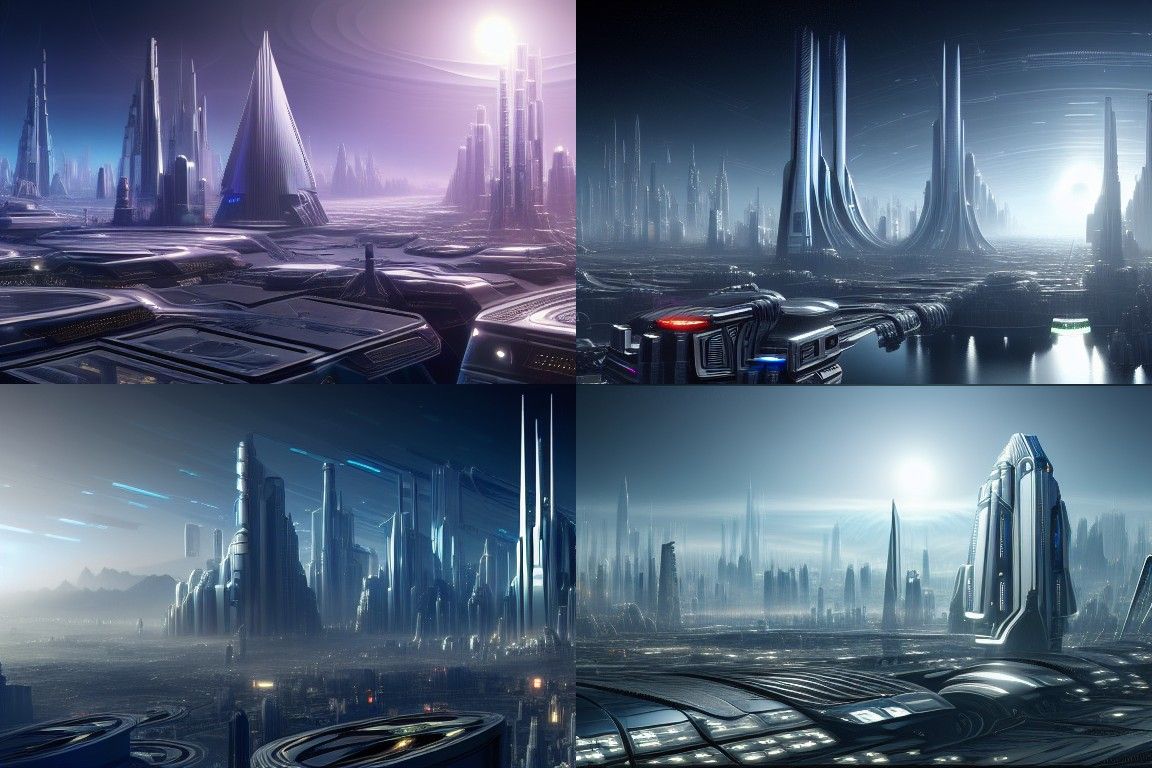The image is divided into four quadrants, all depicting futuristic city scenes that seem straight out of a sci-fi movie, reminiscent of a planet entirely covered by an urban landscape. Each quadrant features prominently tall, uniquely shaped skyscrapers and other massive structures that give a distinctly otherworldly feel.

In the top left quadrant, there is a dominant purplish hue. The scene highlights a large, pyramidal building at its center with a sun casting its light from the background. The top right quadrant presents a more blue-themed cityscape, with towering U-shaped buildings and a militaristic turret in the foreground casting a sense of defense or frontier outpost.

The bottom left quadrant features tall, irregularly shaped buildings set against a backdrop with blue streaks, possibly from vehicles or sky trains, suggesting movement and advanced transportation. Spaceships or aerial vehicles with blue trails are also visible, hinting at a bustling sky traffic system. Finally, the bottom right quadrant, bathed in a lighter blue hue, shows a skyline illuminated by the bright sun. Among its various futuristic buildings, a significant flat structure rises prominently on the right side.

Altogether, the image showcases a high-tech, urbanized world filled with distinctive architecture and advanced machinery, evoking a blend of industrial, militaristic, and cosmopolitan elements in a cohesive sci-fi vision.